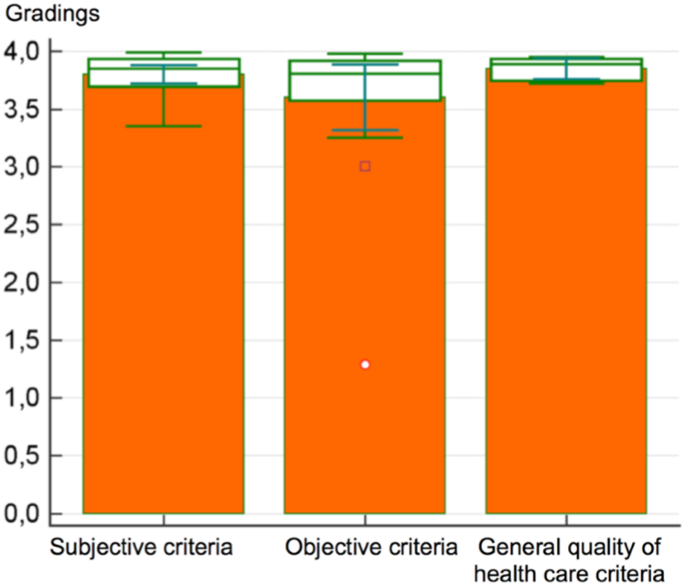The image depicts a bar graph with three wide orange bars representing different evaluation criteria against a GPA scale from 0 to 4.0. The vertical axis, labeled "gradings," is marked with intervals from 0 to 4.0, while the horizontal axis features three labels: "subjective criteria," "objective criteria," and "general quality of healthcare criteria." The leftmost bar for "subjective criteria" stands at approximately 3.75, the middle bar for "objective criteria" at about 3.6, and the rightmost bar for "general quality of healthcare criteria" peaks at around 3.9, making it the highest. Additionally, there are unexplained green lines marking various points on the chart, but no legend is provided. The chart appears to compare GPAs based on different criteria, possibly within an academic context focused on health care quality.